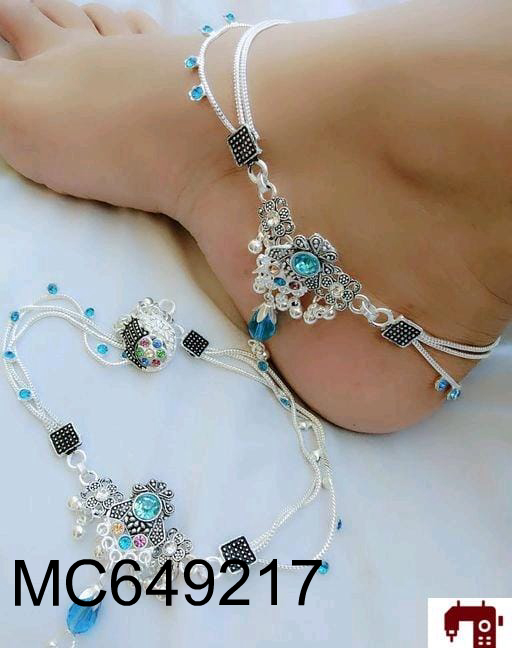This photograph features a detailed view of a woman’s elegantly adorned ankle and foot, partially displaying her toes with the big toe obscured. Her foot is angled towards the upper left-hand corner of the image, with her heel pointing down to the lower right. The foot showcases a highly ornate anklet comprised of three delicate strands of tiny pearl beads, complemented by aquamarine pieces hanging from the lowermost strand. Additionally, there is a silver piece of metal adorned with more aquamarine gems and a striking red ruby, positioned on the inner side of the ankle. The anklet, secured with multiple black charms, features a larger blue gem at its centerpiece and spans around the foot elegantly. The backdrop is a very pale blue, and to the left, another similar anklet with visible chains and gemstones lies flat on the floor. In the bottom right-hand corner of the photograph is a logo depicting a sewing machine and the letters MC649217 printed in black.